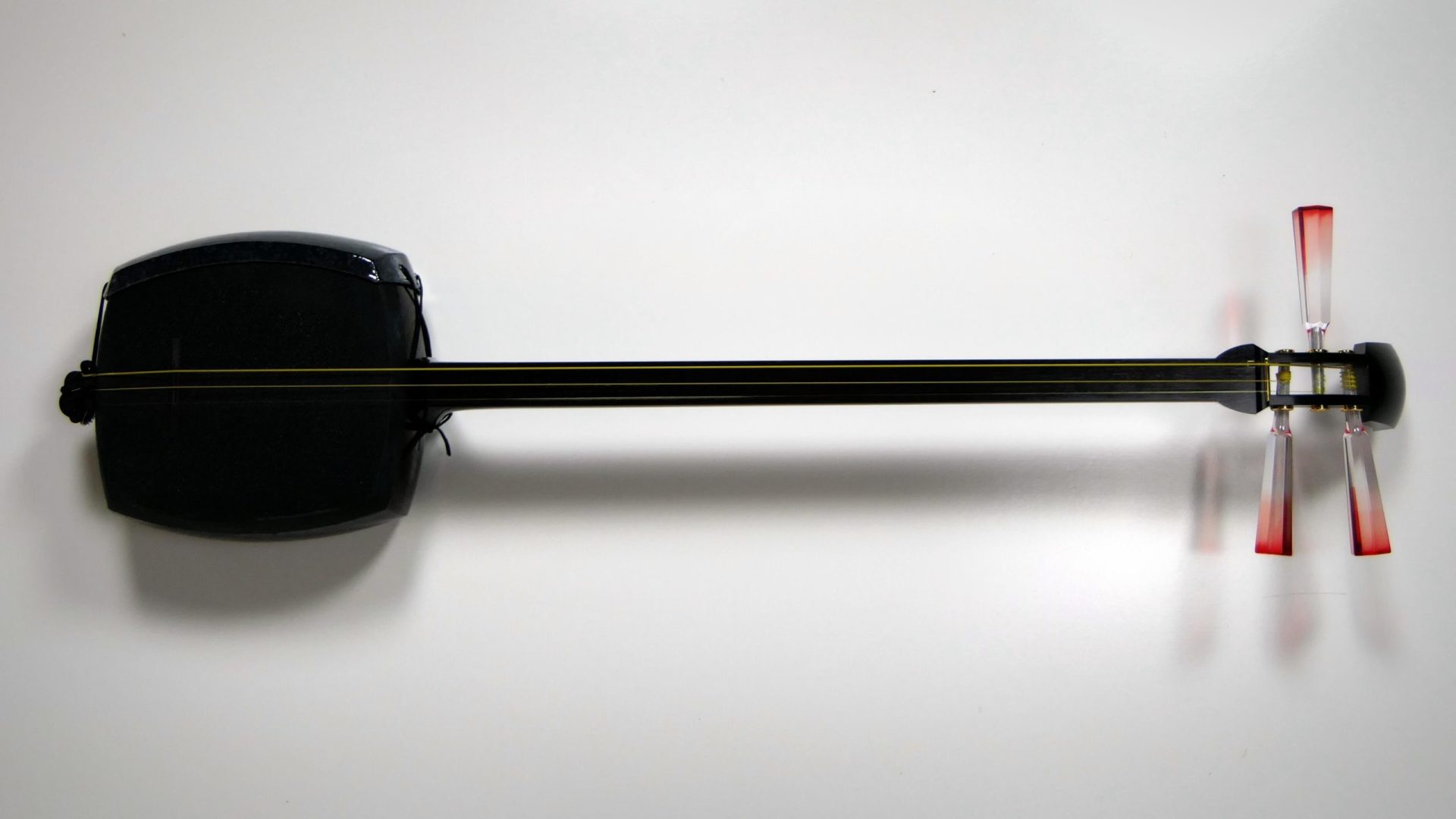This image depicts a detailed view of a traditional stringed instrument, most likely a shamisen. The instrument, oriented with the head to the right, features a glossy black body shaped like a square on the left side of the image. A long, black fretboard extends out from the square body and is fitted with three yellow strings that run across its entire length. At the end of the fretboard, the instrument's head is equipped with three distinct tuning pins: two facing downward and one facing upward. These tuning pins exhibit a gradient of colors, starting from gray and transitioning to a vivid pink before ending in a deep red hue. The instrument is sharply contrasted against a plain white background, with its clear shadow cast behind it.